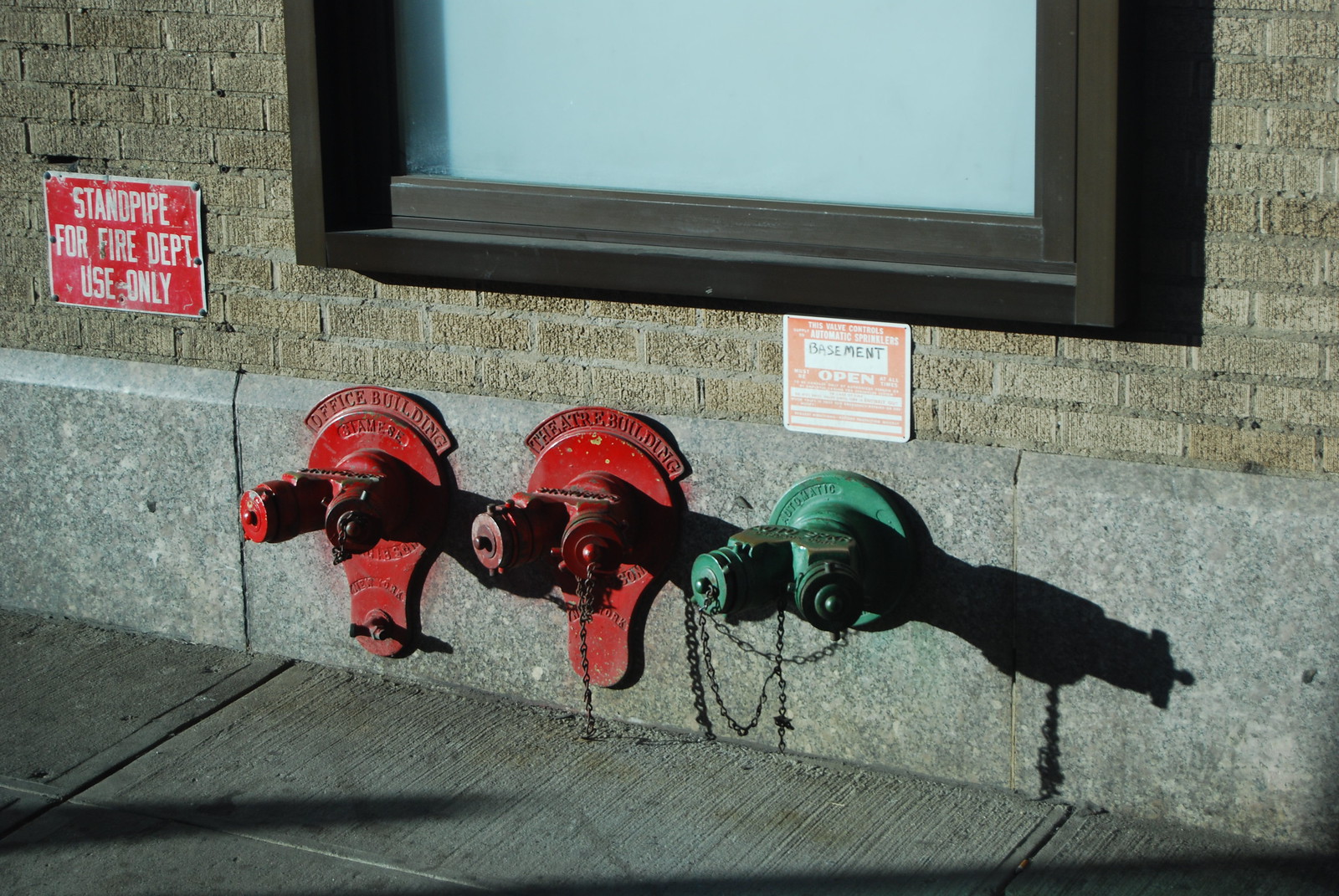This detailed color photograph captures the side of a round brick building with a cement sidewalk in the foreground. The building's facade is composed of light brown bricks with a concrete barrier at the base. Prominently displayed on the left is a red rectangular sign with a white border that reads, "Standpipe for Fire Department Use Only," secured by six fasteners. Below a brown-framed window with white shades is a series of three water pipe assemblies used for firefighting purposes. Each assembly is mounted on cement rectangular plaques. The two on the left are red, labeled "Office Building" and "Theater Building," each featuring two cylindrical valves with smaller central cylinders, and secured with metal chains. The assembly on the right is green, slightly turned, and its label is unreadable. The wall behind the pipes is partly brick and partly smooth concrete, providing a contrasting backdrop to the metallic and colorful fixtures.